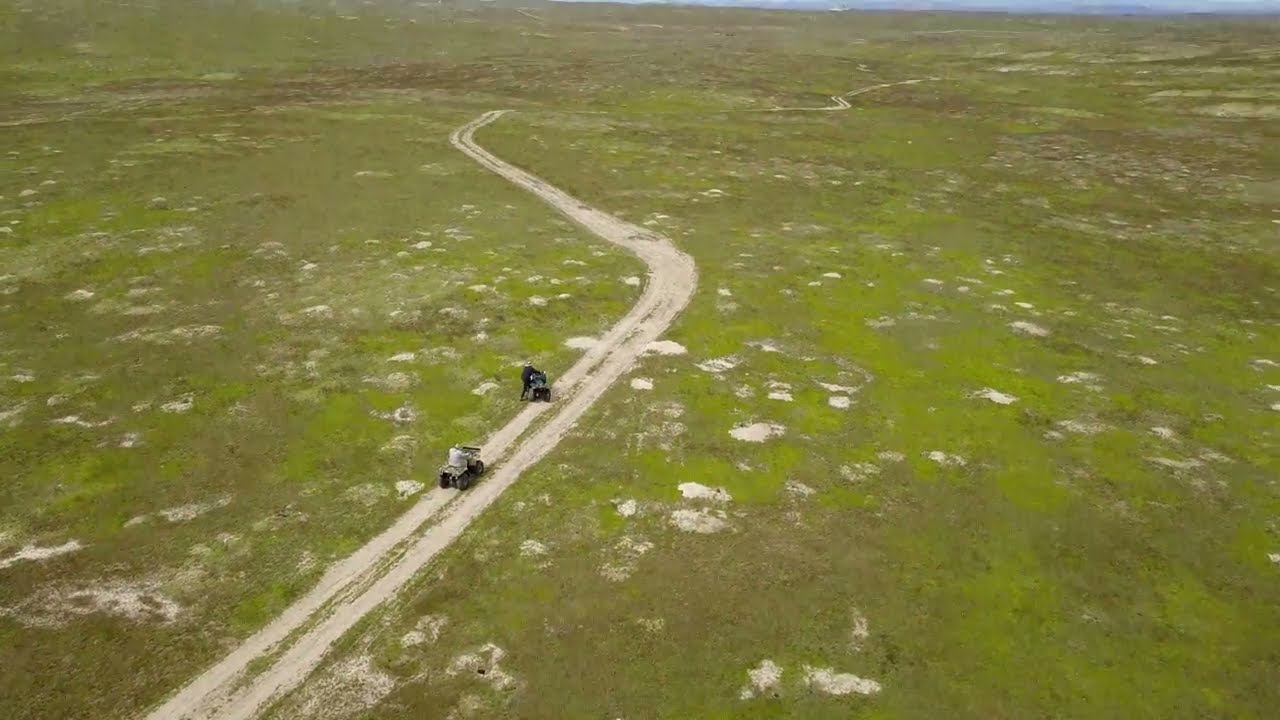The image captures an expansive field, likely used for grazing, with a landscape dominated by vibrant green grass interspersed with patches of grayish-brown vegetation. The bright blue sky is mostly clear, with a few sparse clouds occupying the top 20% of the image. In the lower left corner, a prominent dirt road with heavy grooves starts and travels upward to the mid-right part of the scene. Another less distinct, lightly treaded dirt path branches off this primary road near the right-hand side and winds upward to the left, eventually leading up a hill. A fence lines the lower right section of the image, positioned along the main road. Overall, the setting suggests a tranquil, open area on a clear day, characterized by the contrasting pathways and the expansive, varied grassy terrain.